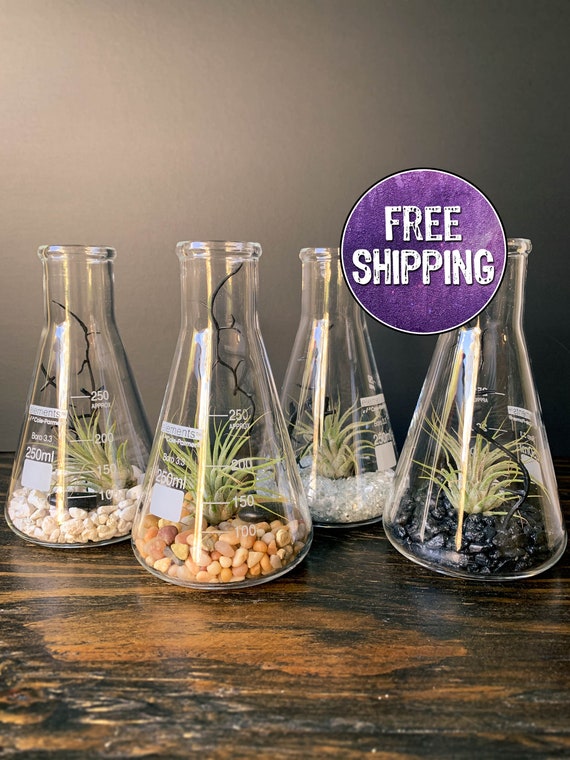The image features four chemistry beakers, each serving as a unique decorative terrarium. They all contain various colored pebbles and vibrant succulents, enhanced by twig-like elements. The beaker on the left is filled with white rocks, while the succulents in the center-left beaker are nestled in brown and yellow pebbles. The center-right beaker showcases white crystal rocks, whereas the beaker on the far right contains black pebbles. All four beakers are arranged on a wooden table against a gray background, with two beakers slightly in front of the others. A purple emblem on the upper right reads "free shipping" in white ink, suggesting an advertisement context.